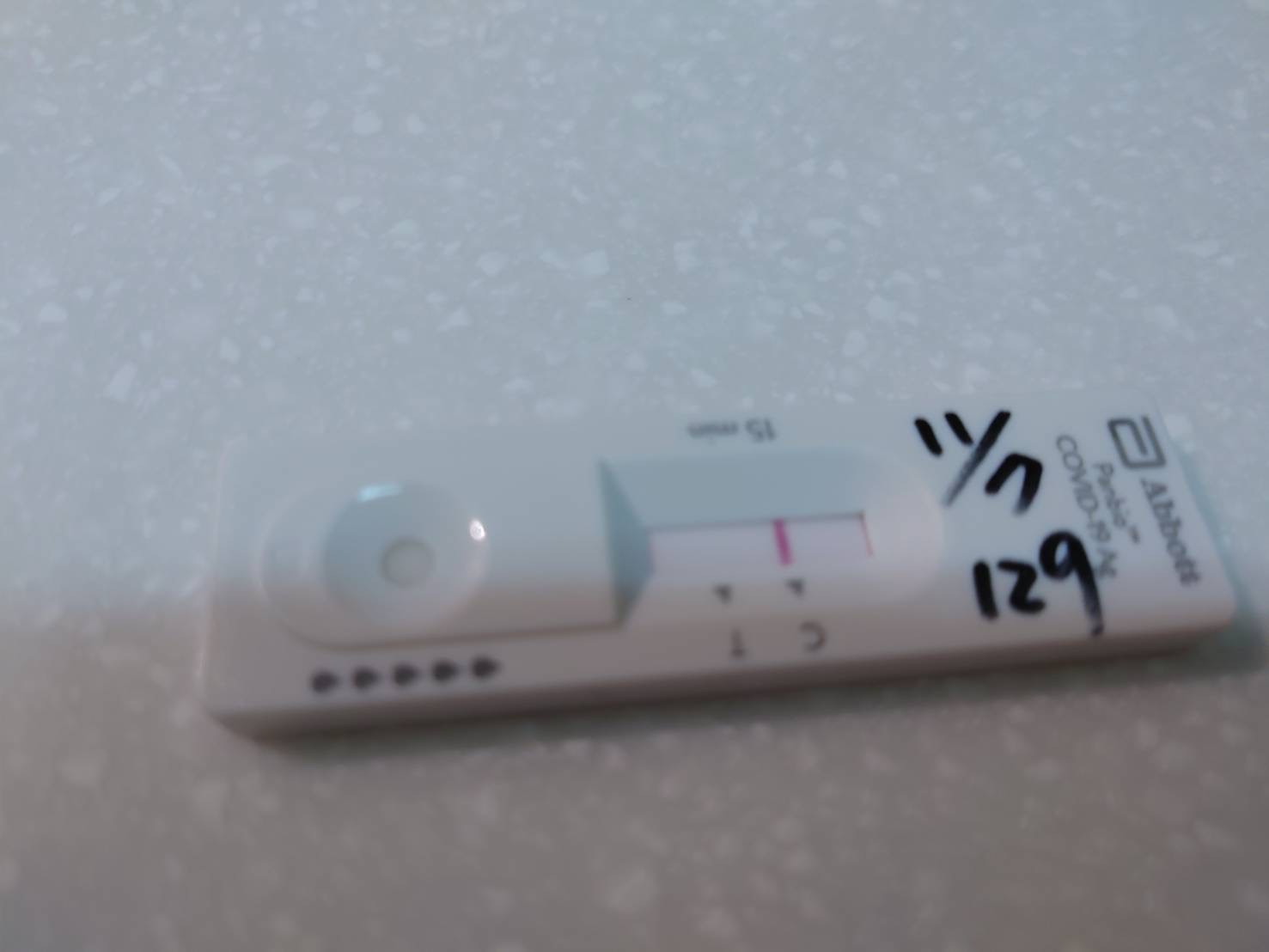This horizontal rectangular photograph showcases a COVID-19 test laid on a white surface with bright white dots scattered throughout. The test kit is positioned slightly lower than the halfway point of the image. The plastic test device itself is predominantly white, featuring branding and text on its right side. At the top of this section, there is a small logo followed by the word "Abbott" in black font with a capital 'A' and lowercase 'b-b-o-t-t'. Directly below "Abbott," the word "COVID-19" is prominently displayed in all capital letters.

The top edge of the test strip has some illegible markings. The bottom edge of the device showcases a complex design. On the left side, there is a raised, semi-circular shape transitioning into a rectangular form with horizontal parallel lines, ending with a vertical line closer to the center. This area is slightly elevated, except for a depressed circular section beneath the semi-circle, which houses a smaller inner circle. Below this circle are five elongated, gray or black dots, with a central depression that mirrors the semicircular shape but in reverse.

On the right side, the semi-circular shape begins on the right, leading into two parallel, horizontal depressed areas, terminating in a vertical line that aligns with the other side. A dark red line is visible vertically beneath an unclear letter in a slightly blurred segment of the test strip. Along the right edge of the test window, a small hint of red can be observed. Additionally, there are handwritten inscriptions in black marker: a notation resembling "11/" followed by something illegible, and below it, the number "129."